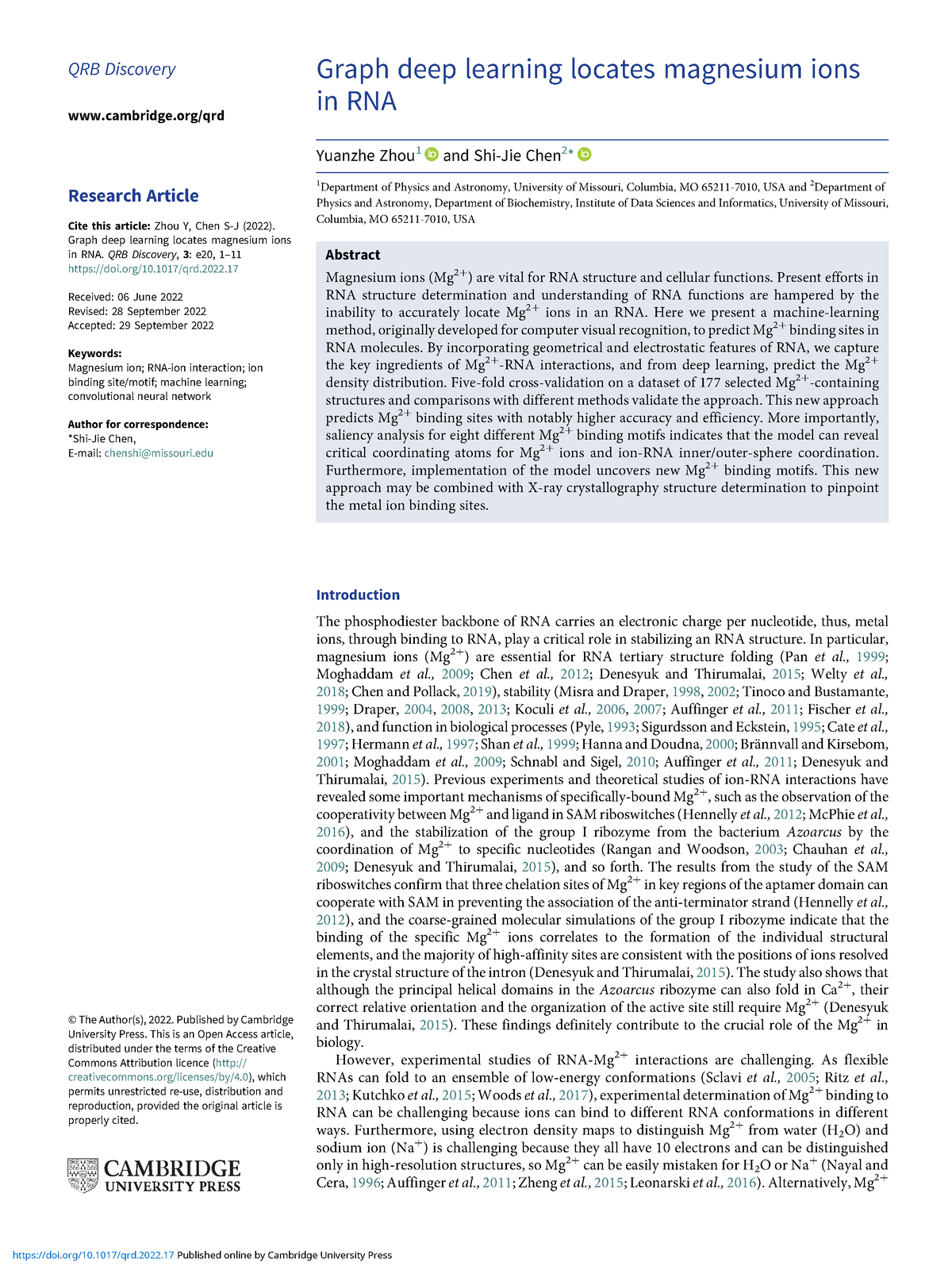**Detailed Caption:**

The image features a research article titled "Deep Learning Locates Magnesium Ions in RNA," published by QRB Discovery. The web address listed is www.cambridge.org/QRD. On the left side of the page, it is clearly labeled as a research article. The article provides the author's name, a list of relevant keywords, and identifies the author for correspondence. Cambridge University Press is credited at the bottom left corner of the page.

Prominently displayed are the contributions of two individuals who spearheaded the research. The introduction section details their departmental affiliations and research context. A highlighted abstract, set within a grey square, states: "Magnesium ions are vital for RNA structure and cellular functions. The current understanding of RNA processes is limited by the inability to accurately locate magnesium ions in RNA." 

The article outlines a new machine learning method adapted from computer visual recognition technology to tackle this challenge. The method is proposed as a novel solution for identifying magnesium ions within RNA structures. The introduction further explains the complex nature of RNA's electronic charge and the importance of metal ions, suggesting that a thorough understanding requires familiarity with specialized terminology.